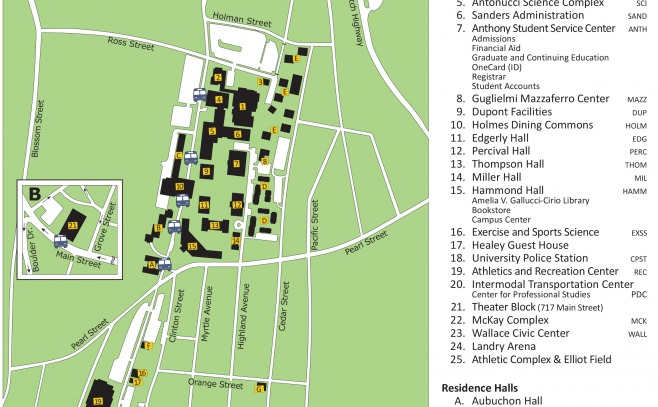This image features a detailed campus map showcasing the layout of a town's university area, including the main buildings and facilities. The map uses a range of colors, including lime green, pale lime green, yellow, black, white, blue, and gray. On the left side, green land is outlined by white roads, which are labeled and numbered up to at least 25, indicating various buildings and points of interest. Key locations are labeled in a mix of black and white outlines, and buildings such as Holmes Diner Commons, Eggerly Hall, Pelvis Hall, Thompson Hall, Miller Hall, Harmon Hall, and the Athletic and Recreational Center are clearly marked. The map also features numbers in yellow rectangles for easy reference. On the right side of the map, descriptive text lists all the buildings and places, providing a comprehensive guide to the campus layout. The close proximity of the labeled buildings suggests a dense, well-organized campus setting, likely serving a smaller university or college community.